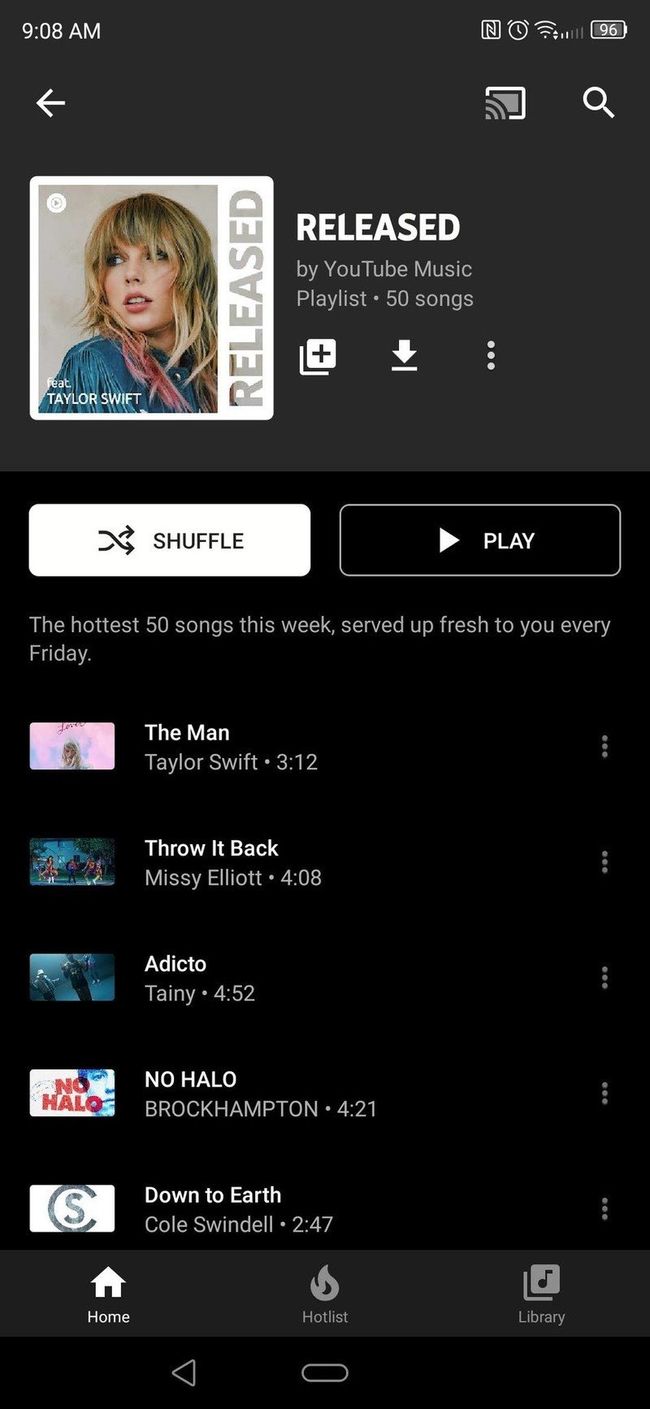Screenshot of a mobile phone displaying the YouTube Music interface in dark mode. The screen shows an album cover featuring Taylor Swift's face and details about a playlist titled "Released" by YouTube Music. The playlist, which includes 50 songs, features the hottest tracks of the week and is updated daily. At the top of the screen, the status bar indicates the time as 9:08 AM, alongside icons for notifications, an alarm clock, Wi-Fi connectivity, and a battery level at 96%. Prominent buttons for 'Shuffle' and 'Play' are visible below the playlist description. Some highlighted tracks include "The Man" by Taylor Swift, "Throw It Back" by Missy Elliott, "Adicto" by Tainty, "No Halor" by Brockham, and "Down to Earth."